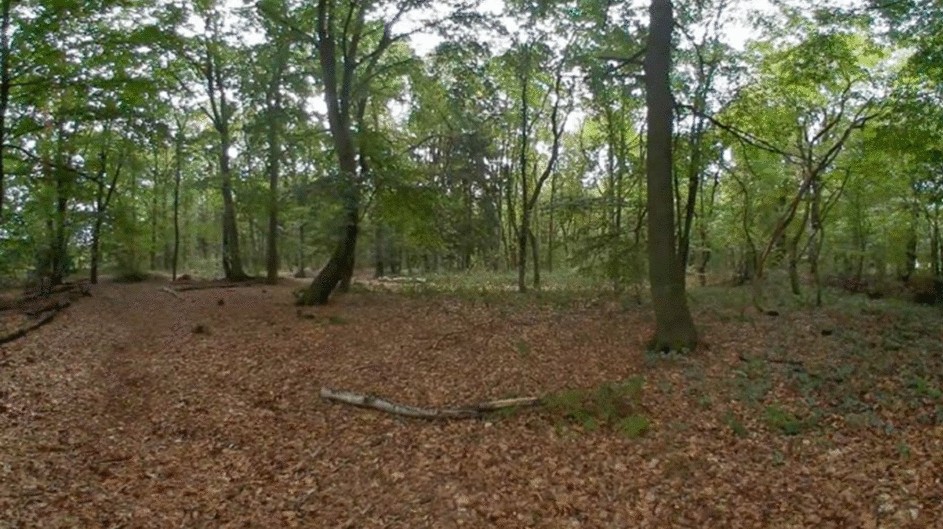The photograph captures a woodland area bathed in daylight. In the foreground, there's a clearing blanketed with a thick layer of dead leaves and dirt, adding to the notion of minimal sunlight reaching the ground. A prominent, large, barren tree branch lies diagonally across the center of the clearing, devoid of any leaves. Surrounding the clearing, the dense forest is rich with green foliage, suggesting it is a season of lush growth. The background is filled with a multitude of trees, providing a stark contrast between the vibrant, thick canopy above and the scattered, leaf-covered ground below. Light peeks through the gaps in the tree canopy, illuminating patches of the forest floor and highlighting the chaotic, untamed nature of the woods. The scene is devoid of any human presence, emphasizing the wild, serene quality of this forest landscape.